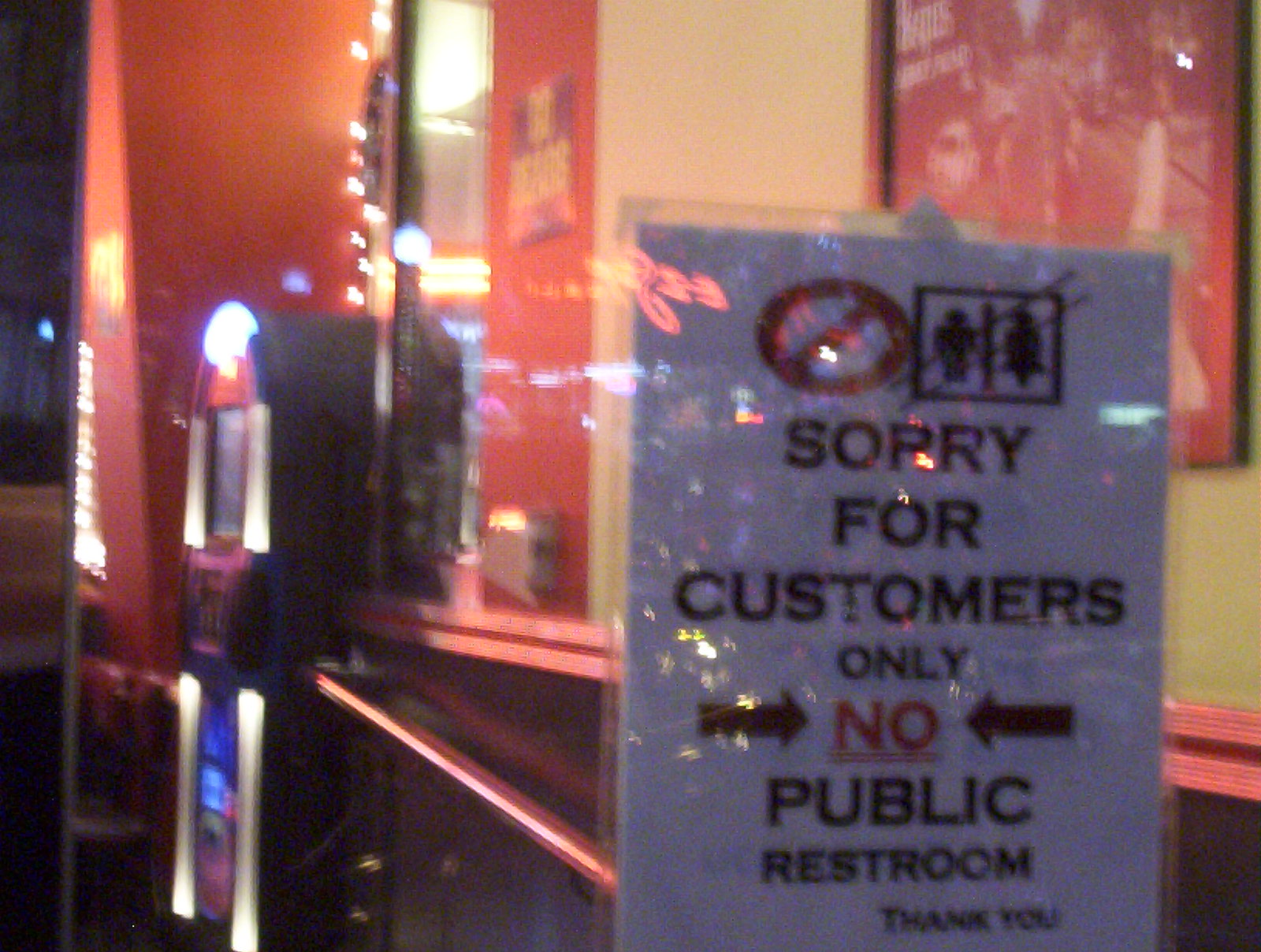In this blurry nighttime photo, shot through a reflective glass window, the foreground prominently features a laminated sign with a red circle and a line crossed through bathroom icons, indicating, "Sorry for customers only, no public restroom, thank you." The sign reflects colorful street lights, adding shiny reflective colors to it, with hues of purple, gray, and yellow intertwined. Beyond the sign, the image captures the blurred interior of a store. Cream-colored walls frame a red poster adorned with white text and additional red and orange elements. On the right side, another sign with a purple background and yellow writing is barely readable due to the blur. Strewn lights can be seen outside, hanging by black wires. The left side of the photo hints at a green-lit traffic signal and a transitioning blue-to-black sky, emphasizing the onset of night. The road outside appears gray with yellow lines. In the middle of the scene, possibly an ATM is noticeable with white, red, and yellow illuminated sections, adding to the nighttime ambiance.